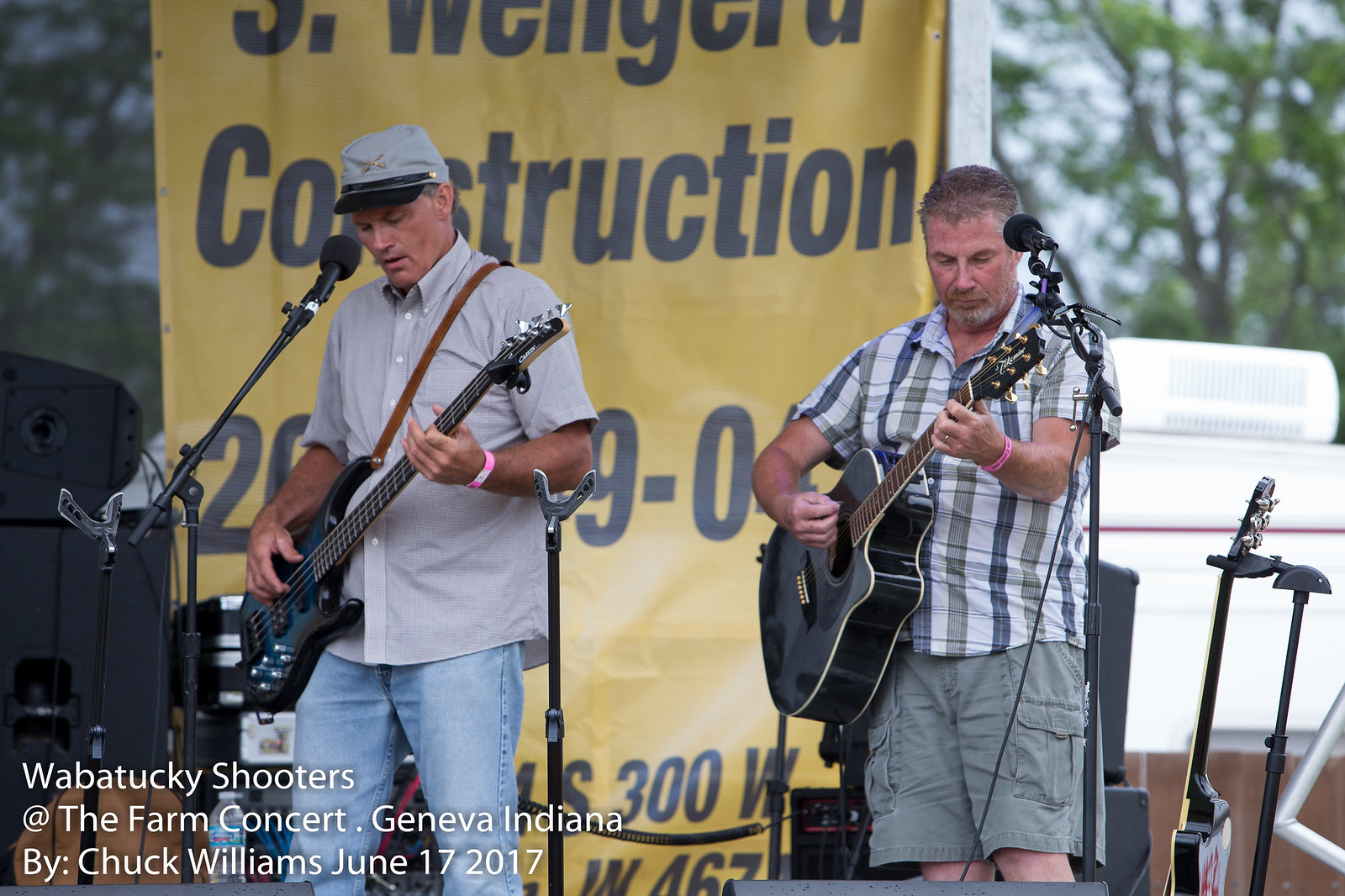This picture captures a daylight outdoor concert featuring the Wabatuckee Shooters at the Farm Concert in Geneva, Indiana, on June 17, 2017, as documented by Chuck Williams. Two white male musicians are on the stage. The gentleman on the left is playing a black electric guitar, wearing a light gray short-sleeved shirt, blue jeans, and a gray cap with a black bill. He stands in front of a microphone on a stand, singing into it. To his left, there's another empty mic stand and a water bottle near his knee level. His bandmate on the right is playing a black or dark gray acoustic guitar while wearing a white, short-sleeved button-up shirt with a black and gray striped pattern and gray cargo shorts. He has salt-and-pepper hair and a matching beard, also performing in front of a microphone stand. Both musicians have entry bands on their left wrists. In the background, an upright guitar rests against a post and additional musical equipment, including speakers and boxes, are visible. A large, partially visible yellow banner with black lettering hangs behind them, advertising "Wangler Construction" with some partially obscured numbers and an address. Trees and an RV can be seen further back, enhancing the outdoor ambiance.